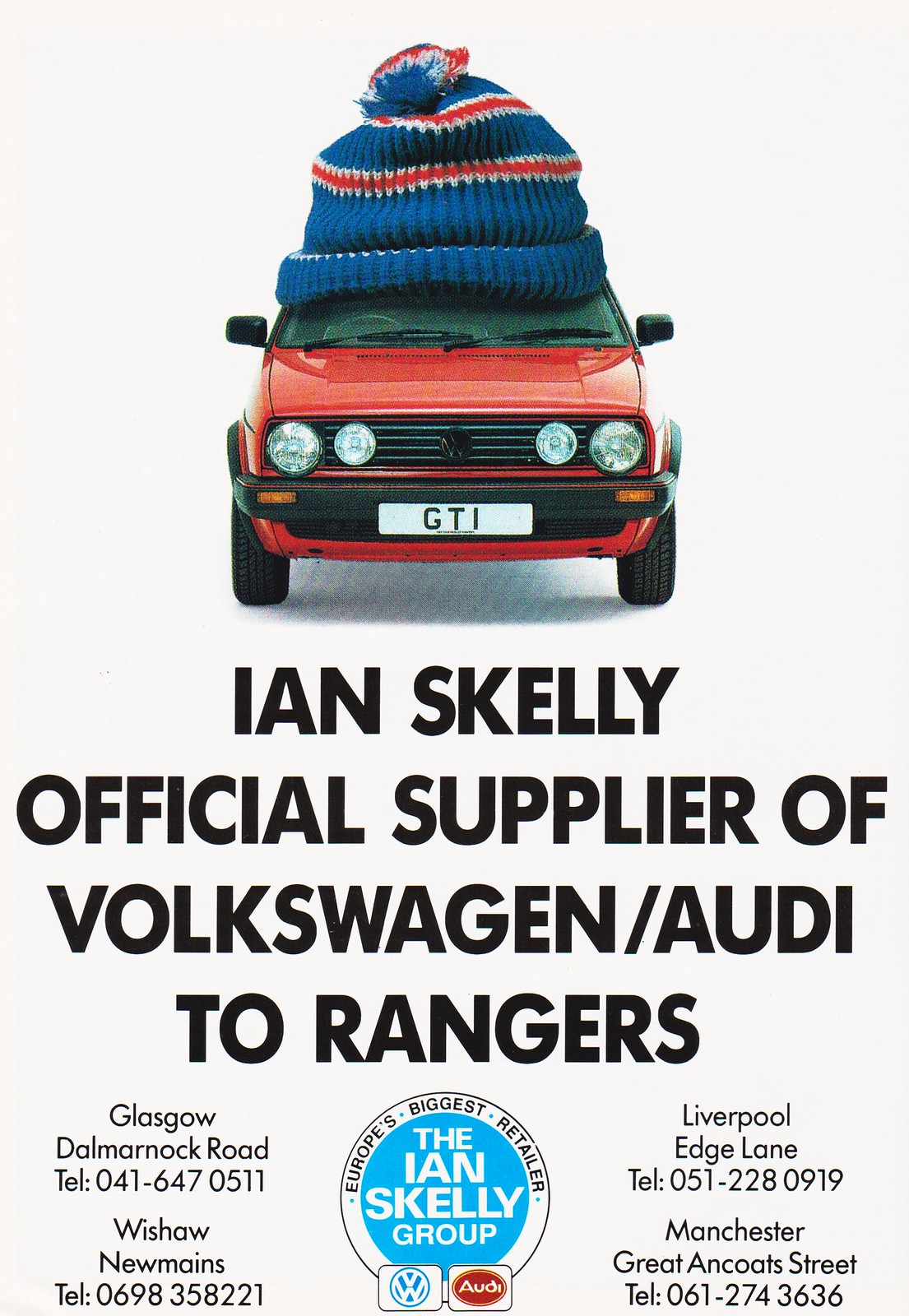This vertically aligned advertisement features the front of a red Volkswagen GTI adorned with a whimsical, oversized blue beanie with red stripes and a multi-colored pom-pom on top. The backdrop is a light gray, emphasizing the vibrant car and its quirky hat. Below the car, in bold black letters, it reads: "Ian Skelly, official supplier of Volkswagen/Audi to Rangers." Four contact locations are detailed at the bottom—Glasgow, Wishaw (New Mains), Liverpool (Edge Lane), and Manchester (Great Ancoats Street)—with corresponding telephone numbers. Centrally, between these contacts, is a blue circle logo with white text that says "The Ian Skelly Group." The advertisement aims to highlight the dealership's association with Volkswagen and Audi, offering a playful yet informative presentation.